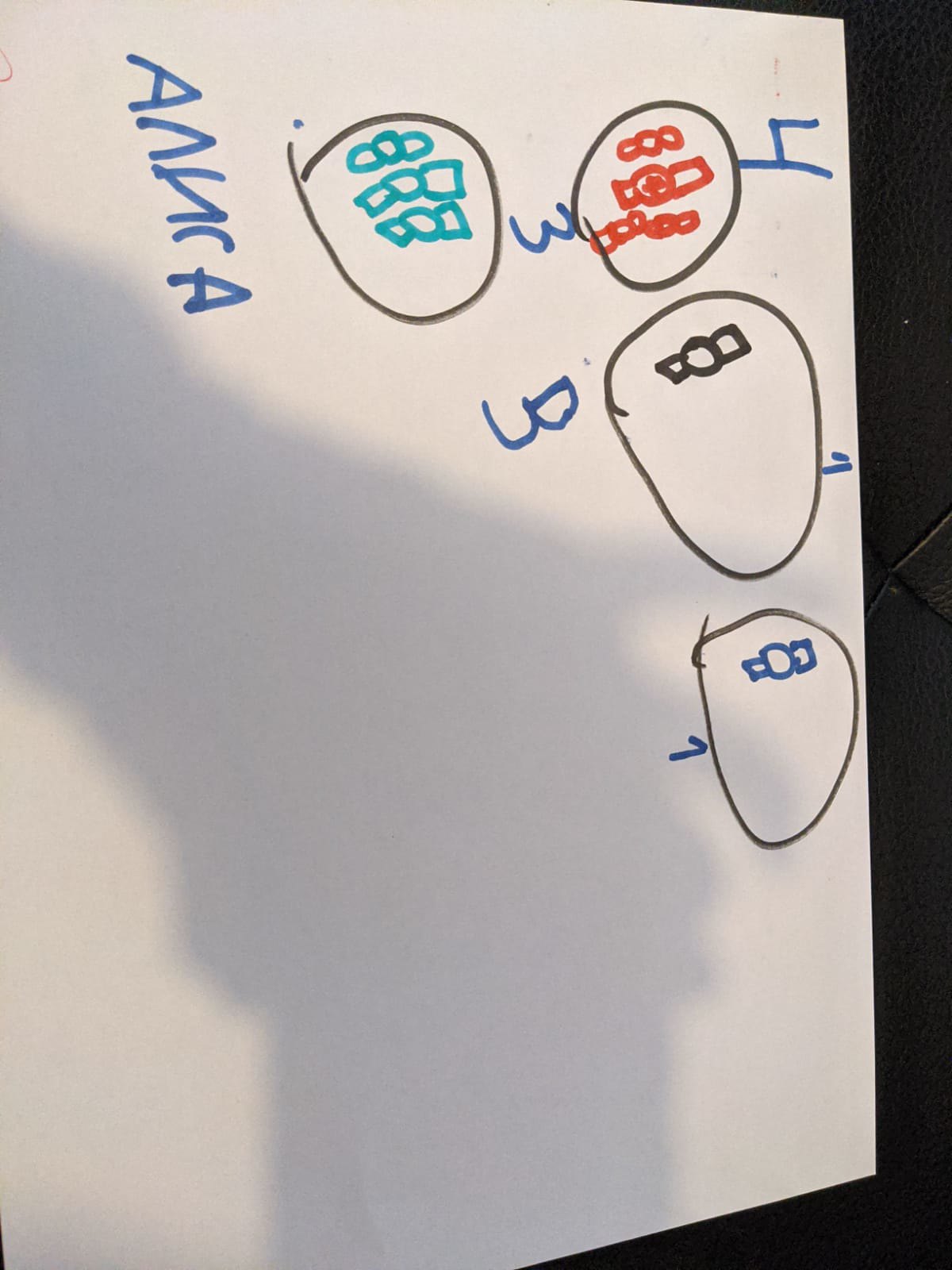In this portrait-oriented image, we observe a sheet of white paper adorned with a colorful assortment of magic marker drawings, likely the imaginative creation of a child. On the right-hand side, three roughly sketched circles are vertically aligned from top to bottom. The top circle, outlined in black marker, contains intersecting circles in a chain-like pattern and two squares flanking a central circle, all rendered in red marker. The middle circle, also in black, encloses a small circle and two adjoining squares near its upper section. The bottom circle, distinguished by its egg-like shape, features a small circle and two squares, all drawn in blue marker.

Positioned in the upper central region of the page is another black circle, populated with three configurations, each consisting of a circle accompanied by small adjoining squares, meticulously depicted in aqua marker.

Along the left margin of the page, we see roughly inscribed letters in blue marker, which apparently spell out the name "Anna," though the clarity is compromised. A gray, irregularly-shaped shadow casts across the paper, adding a touch of depth to the image.